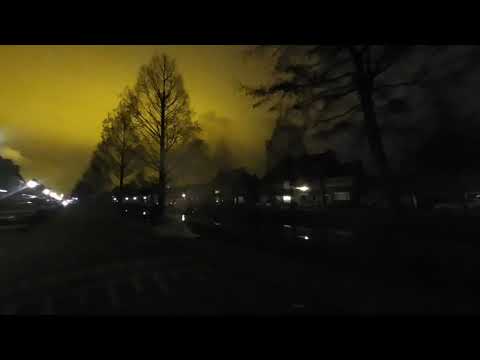This image captures a night scene characterized by a dark and shadowy atmosphere, accentuated by a striking yellow, golden-rod colored sky. Silhouettes of several houses and deciduous trees without leaves stand out against the backdrop. The houses, lined along a road in the center of the image, feature white lights glowing through their windows, piercing the surrounding darkness. The trees near the top of the image appear tall and barren, adding to the eerie nocturnal setting. The bottom half of the photograph is enveloped in deep shadow, rendering it difficult to distinguish any specific details. The overall image borders at the top and bottom, framing this quiet, dimly lit outdoor scene.